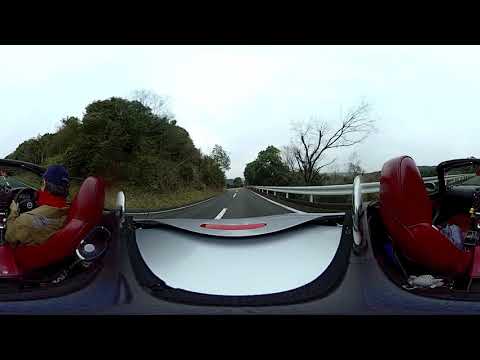This panoramic or fisheye image captures a unique view from within a convertible vehicle. The distortion makes it challenging to pinpoint the exact vehicle shape, but it features two bright red bucket seats—one on the left with a driver and an empty one on the right. The driver, clad in a light brown or beige jacket, a red scarf, and a blue cap, has his hands on a black steering wheel. A metallic gray element likely representing the vehicle's body connects the two seats. 

Behind the vehicle, stretches a two-lane dark gray asphalt highway lined with white stripes and a guardrail on the right, safeguarding from what appears to be a drop-off flanked by trees. On the left side of the road, the ground rises gently, covered with grass and dotted with shrubs and fluffier trees. The sky above has an overcast, pale bluish-gray hue with clouds, lending an otherworldly turquoise tint to the scene. The image provides a surreal yet picturesque snapshot of a roadside landscape framed by black borders at the top and bottom.